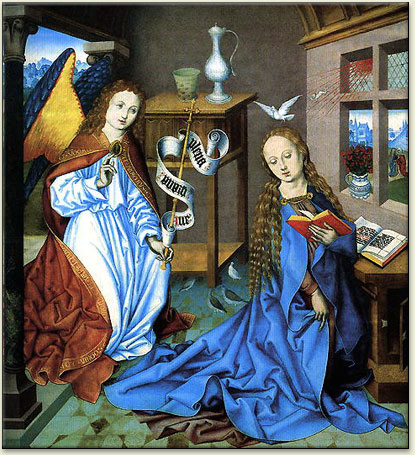The image depicts a detailed scene of a woman and an angel set within a medieval environment. Central to the composition is a young woman with long, braided brown hair cascading past her waist. She is seated at a desk or table, engrossed in reading a red book held in her left hand, while her right hand gracefully gathers her blue cloak, which drapes elegantly to the floor and over the rug beneath her. Above her head, a white dove perches quietly.

To her right stands an angel, characterized by long, curly brown hair and a serene expression. The angel is dressed in a whitish-blue gown and a brick red cape, and wields a staff adorned with a winding banner that culminates in a cross. The angel's wings are a striking combination of gold and blue, adding a celestial glow to the scene. With her right hand raised as if offering a blessing, she appears to be bestowing guidance upon the woman.

The setting is ornate and medieval, featuring a green and brown marble floor that complements the intricate arched doorway through which the angel entered. Behind the figures, a table holds a vase and a lamp, adding to the scene's domestic tranquility. To the right, an open window framed in gray lets in soft light, casting gentle shadows on a nearby table that holds another open book. This tableau combines elements of religious iconography and classic medieval artistry, creating a rich and vividly detailed narrative scene.